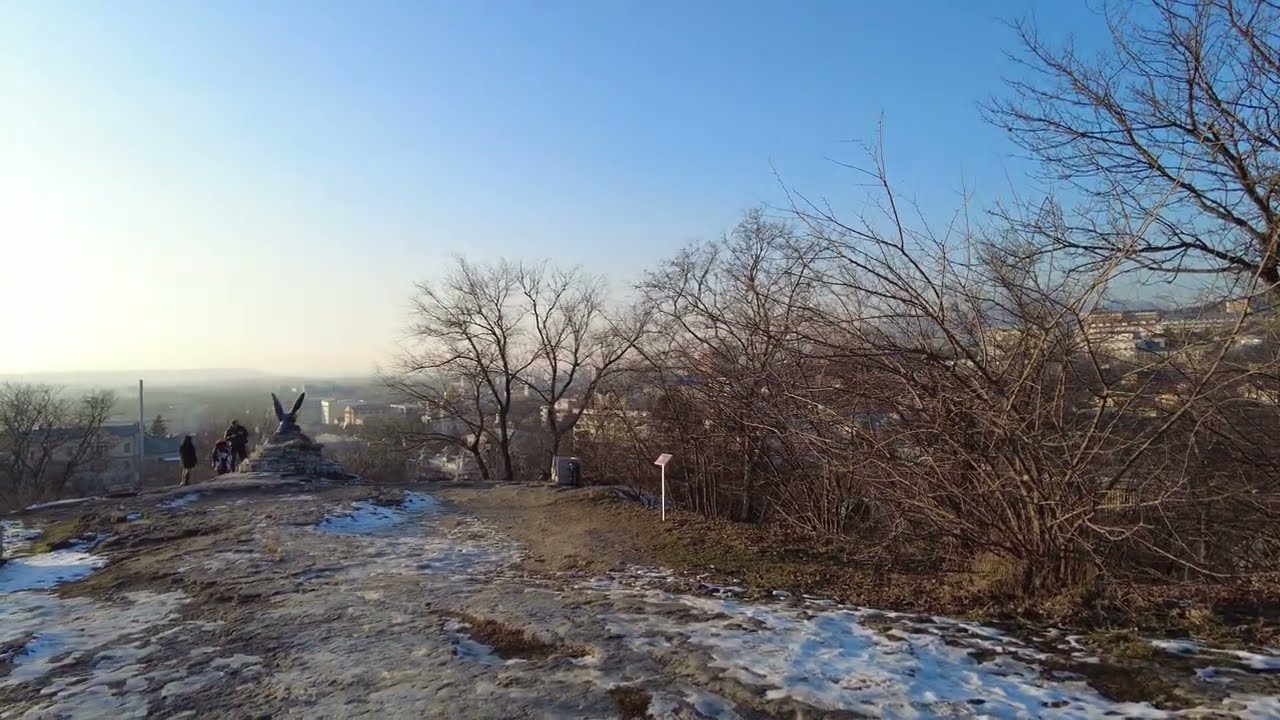The photograph showcases a picturesque scene taken from an elevated hilltop. The upper third of the image features a stunning blue sky with a faint white hue on the left side, likely indicating the sun's presence. The foreground consists of a mix of brown dirt and patches of lingering snow, capturing the raw, rugged terrain of the hill. Scattered across this ground are various puddles, leaves, and sticks, typical of a late fall or early winter setting. To the right and left of the hill's edge, there are several leafless, winter-stricken trees. In the distance, the view opens up to a sprawling valley dotted with building structures. A notable feature on the left side of the hilltop is a winged cement statue-like structure, near which three people can be seen standing, adding a sense of scale and human presence to the landscape. The entire scene is bathed in natural light, offering a serene yet somewhat desolate atmosphere.